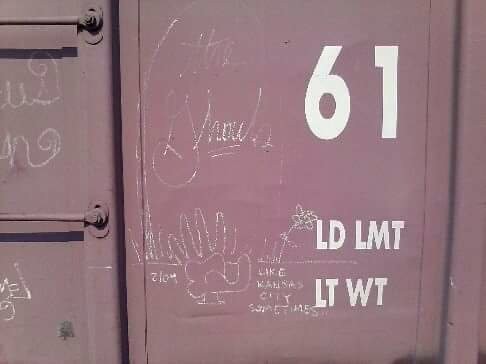This photograph is a close-up of a weathered, rusty red cargo container or railcar, showcasing numerous details. Prominently displayed in the upper right-hand corner are white stenciled letters and numbers, with the number “61” at the top, followed by “LDLMT” and “LTWT” below it. On the left side of the container, two metal rungs of a ladder are visible. The surface is adorned with chalk-like graffiti, including the phrase “Kansas City sometimes,” a flower, and a hand drawing, among other indistinct script markings. The backdrop, a mixture of a dusty pink and grayish surface, adds to the gritty, industrial aesthetic of the scene.